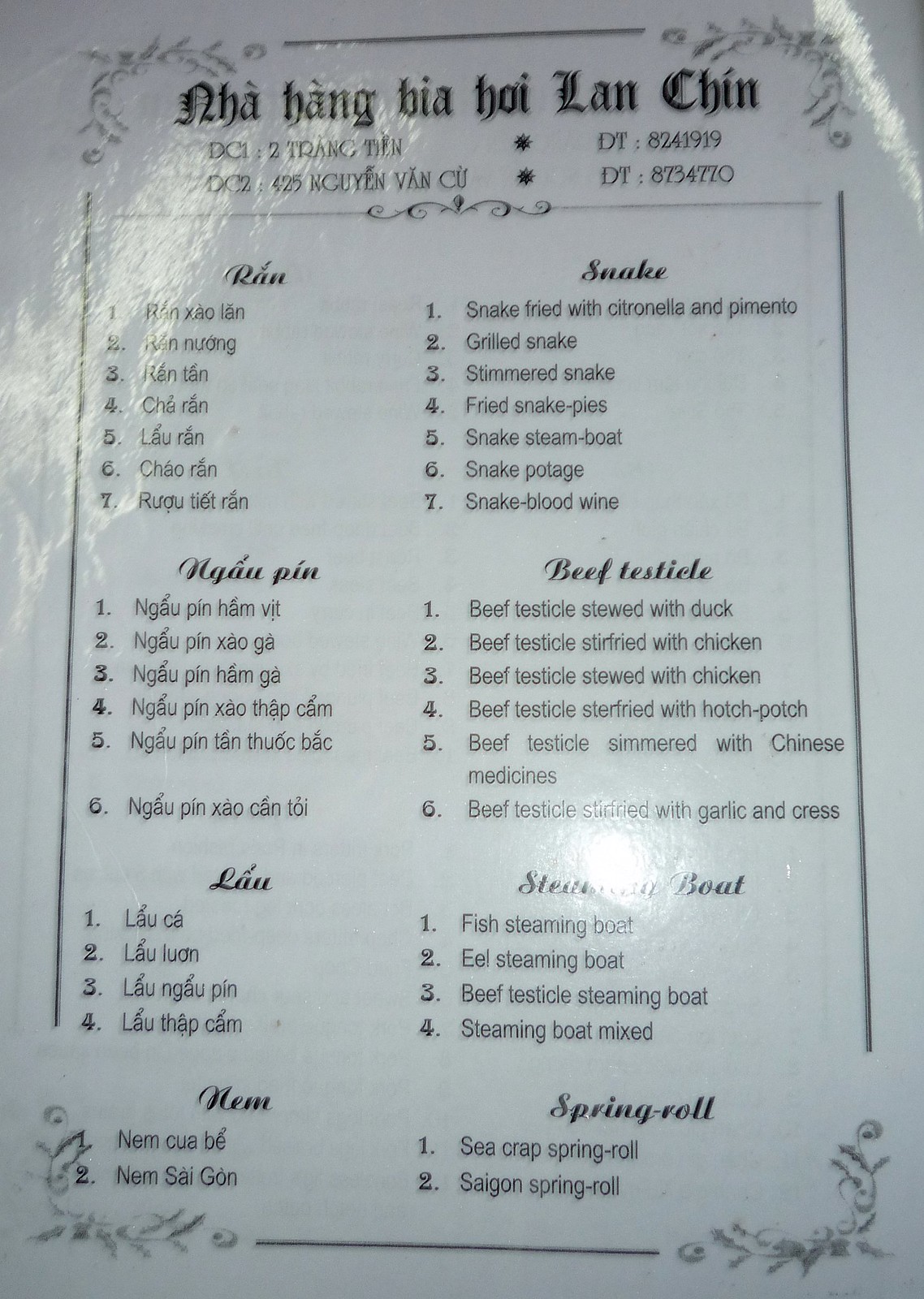The image features a detailed menu from a restaurant, occupying the entirety of the frame from top to bottom. The menu has a white background and appears to be laminated, as evidenced by prominent light reflections on the top left, top right, and bottom middle right sections. The text is in black, with a decorative floral design adorning each of the four corners: top left, top right, bottom left, and bottom right.

At the top of the menu, the restaurant's name is displayed in a foreign language. Midway down the left side of the menu, the section titled "RAN" is prominently highlighted in bold black text. Under this heading, a list of items numbered 1 through 7 extends vertically, each paired with non-bolded descriptions: RAN-ZAL-LAN, RAN-NU-RING, RAN-TAN, SHA-RAN, LA-RAN, and SHAO-RAN.

On the middle right side, another section is distinctly marked with the bolded black word "SNAKE". This section also features items numbered 1 through 7, each with detailed descriptions next to them: 
1. SNAKE FRIED with CITRINAL and PIMENTO
2. GRILLED SNAKE
3. SIMMERED SNAKE
4. FRIED SNAKE FRIES
5. SNAKE STEAM BOAT
6. SNAKE POTTAGE
7. SNAKE BLOOD WINE

The menu presumably continues in a similar format, with various sections featuring different culinary offerings, each neatly organized and descriptive.